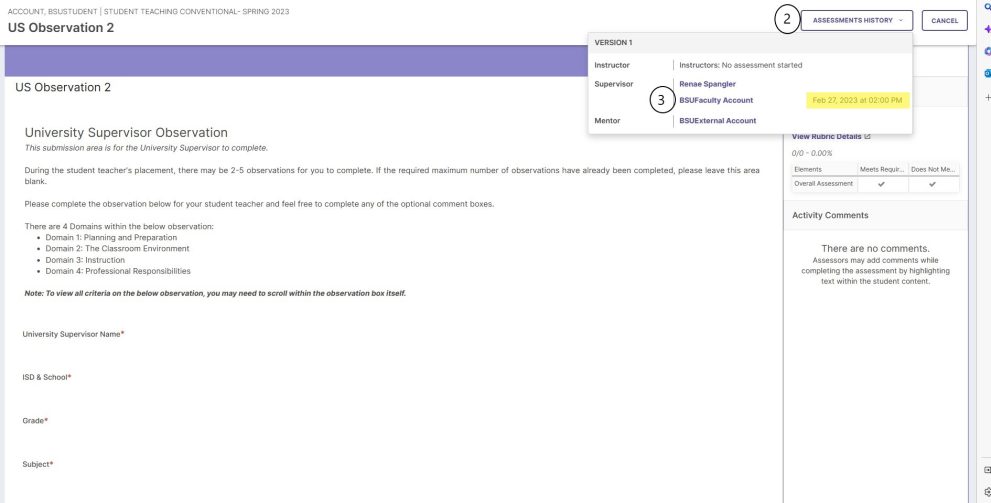Screenshot of a University Supervisor Observation Form on a Website, Spring 2023

In this screenshot, the top left-hand corner of the webpage features a header reading, "Account: Student Teaching, Conventional Spring 2023." Directly beneath that, the text "U.S. Observation 2" is prominently displayed. To the far right on the same line, a circular icon with the number "2" is visible, followed by the label "Assessment History" within an open drop-down menu. This drop-down menu includes options such as "Version 1," "Instructor," "Supervisor," and "Mentor." Adjacent to this menu is a "Cancel" button.

In the main content area on the left side of the screen, the heading "U.S. Observation 2 - University Supervisor Observation" appears. The submission area is designated for the university supervisor's use. Below this, a detailed message explains the observation process, stating: "During the student teacher's placement, there may be two to five observations for you to complete. If the required maximum number of observations has already been completed, please leave this area blank. Please continue the observation below for your student teacher and feel free to complete any of the optional comment boxes."

The observation form is divided into four domains: 
1. Planning and Preparation
2. The Classroom Environment
3. Instruction
4. Professional Responsibilities

A note advises users that to view all criteria within the observation box, they may need to scroll within it. Fields for "University Supervisor Name," "ISD and School," "Grade," and "Subject" are present. 

On the right side of the screen, there is a comment box partially obscured by the drop-down menu, making the top portion of the comment text unreadable.